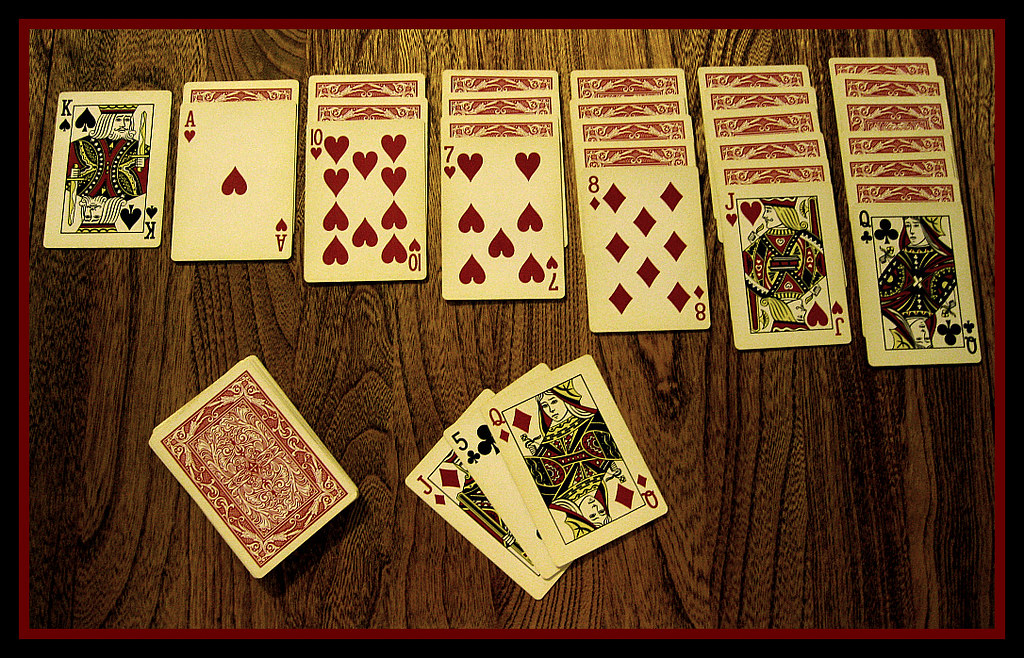A photograph captures a meticulously arranged solitaire game on a dark, wood-grained table. The tableau consists of seven stacks of playing cards, each staggered with one card partially covering the one beneath it. From left to right, the stacks are as follows:

1. A single King of Spades.
2. An Ace of Hearts with one face-down card behind it.
3. A Ten of Hearts with two cards behind it.
4. A Seven of Hearts with three cards behind it.
5. An Eight of Diamonds with four cards behind it.
6. A Jack of Hearts with five cards behind it.
7. A Queen of Clubs with six cards behind it.

In front of these stacks are three more cards laid out: a Jack of Diamonds, a Five of Clubs, and a Queen of Diamonds. To the far right is a deck of face-down cards featuring a red pattern on their backs. This distribution suggests an ongoing game of solitaire, illuminated by the rich texture of the wooden table beneath. The photograph hangs on the wall like a piece of art, capturing the beauty and strategy of the classic card game.